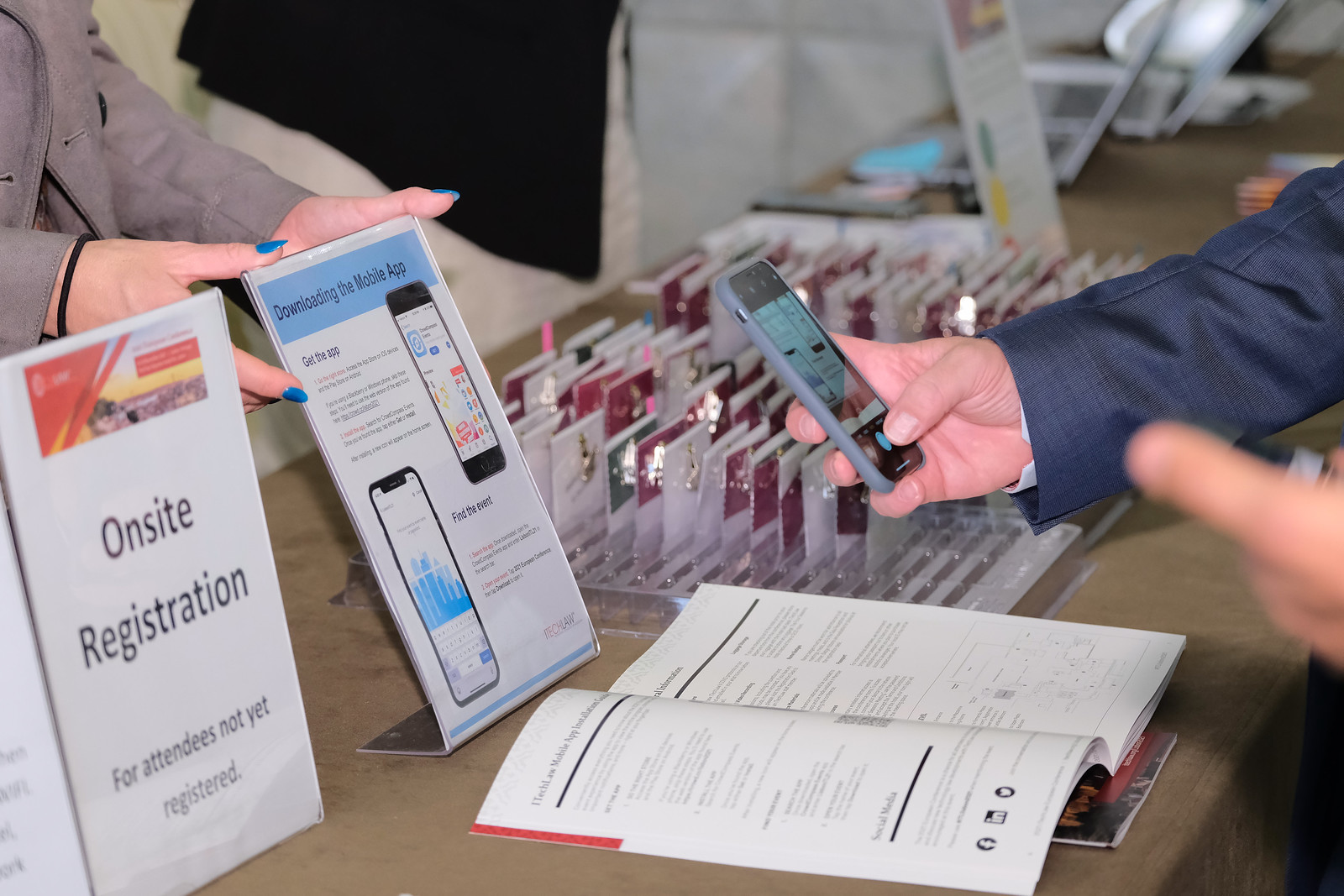In the image, a well-dressed man in a navy suit is captured mid-action as he holds his phone over a wooden desk, seemingly taking a photo or video of a sign. The sign, held by a woman's hands adorned with blue nail polish, reads "Downloading the Mobile App" and has images of two mobile phones with accompanying text instructing how to get the event's app. Another sign on the desk states "On-site registration for attendees not yet registered." On the desk, which resembles a counter at an event or store, various items are scattered, including an open magazine, books, pamphlets, plastic cards in a container, and additional signs and advertisements. The backdrop is a mix of black with a white banner, framing the exchange of information between the two individuals centered around the event's digital resources.